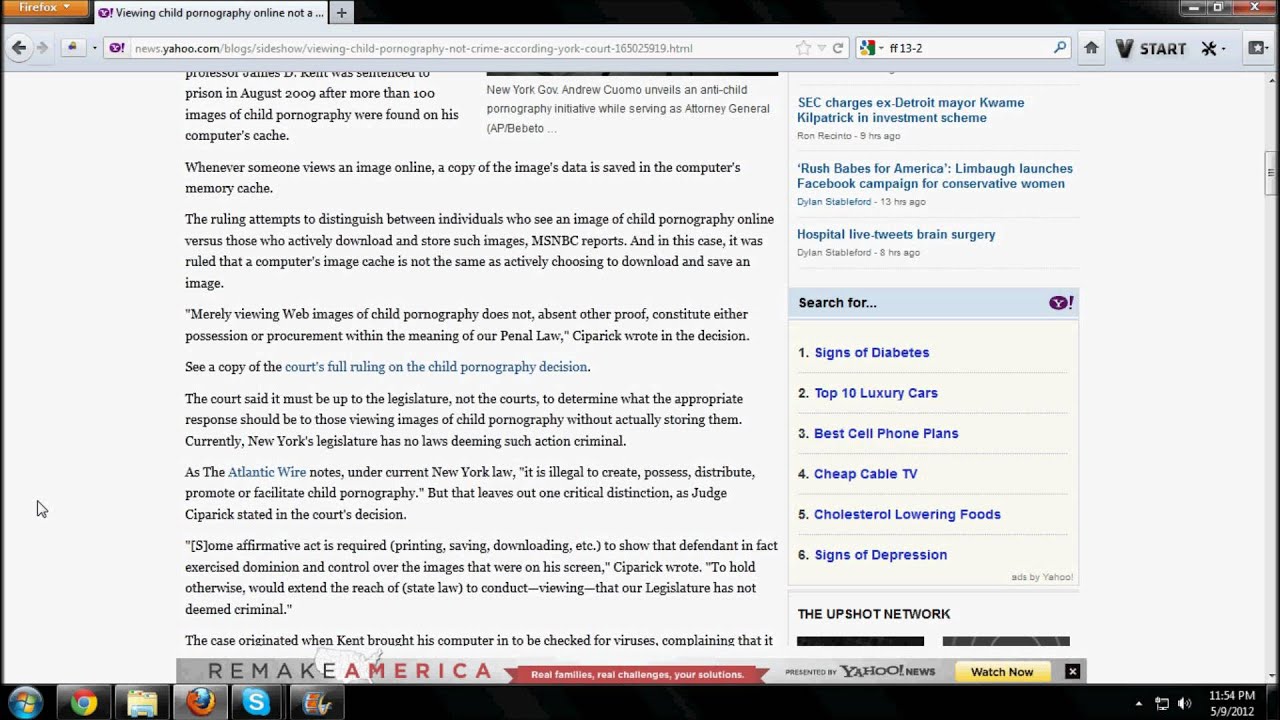Here is a more organized and detailed caption based on the provided information:

---

In this image, we see a screenshot of a website displayed in the Firefox browser. The address bar contains the URL "yahoo.com/blog/site," and the webpage features an article with a striking headline: "Viewing Child Pornography Not a Crime According to New York Court." 

The article elaborates on a recent court decision which differentiates between merely viewing an image of child pornography online and actively downloading or storing such images. According to the ruling, when someone views an image online, a copy of the image data is temporarily saved in the computer's memory cache. The court determined that this involuntary data caching does not equate to actively choosing to download and save an image. 

Judge C. Patrick, in his decision, articulated that merely viewing images of child pornography does not, absent other evidence, constitute possession or procurement under the current penal law. He emphasized that whether viewing such images without storing them should be criminalized is a matter for the legislature, not the courts, to decide. Currently, New York legislation criminalizes the creation, possession, distribution, promotion, or facilitation of child pornography, but it does not address the act of viewing without additional affirmative actions like printing, saving, or downloading.

The case that led to this ruling originated when an individual named Kent took his computer for a virus check and certain suspicious activities were discovered. The article cuts off at this point but provides insight into the nuanced legal distinctions being made in this domain. 

At the bottom of the webpage, a banner advertises “Remake America: Real Families, Real Challenges, Their Solutions.” On the right sidebar, there are various search suggestions including topics such as "Signs of Diabetes," "Top 10 Luxury Cars," "Best Cell Phone Plans," "Cheap Cable TV," "Cholesterol Lowering Foods," and "Signs of Depression."

---

This caption aims to encapsulate the complexity and content of the displayed webpage in a structured and detailed manner.